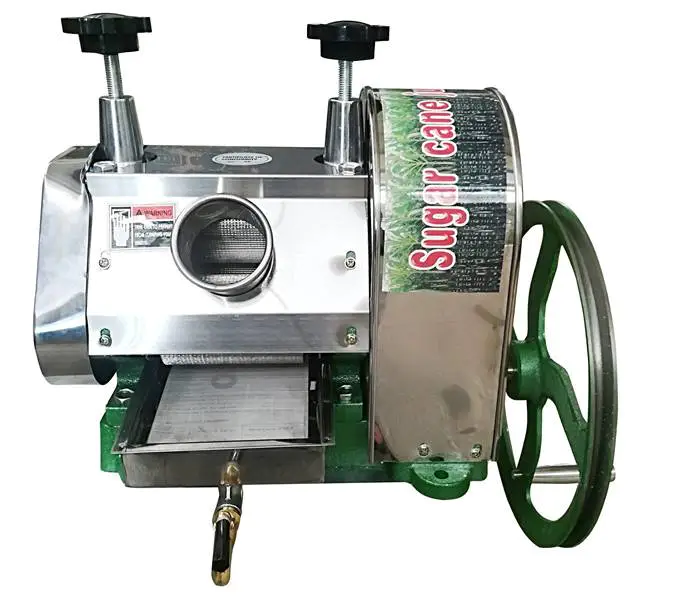The image displays an older, farm-style sugar cane juice extraction machine, primarily constructed from stainless steel with a silver finish. The apparatus features an opening in the middle for feeding sugar cane stalks into the machine. At the top, there are two threaded black adjustment knobs, presumably used for adjusting the spacing between the rollers that squeeze the juice from the cane.

On the right side of the machine, there is a green crank wheel that can be manually turned to operate the juice extraction process. This wheel could potentially be connected to a motor via a fan belt for automated operation. The machine is adorned with a large sticker reading "sugar cane" in red type, with an illustration of sugar cane stalks in the background, although the text is partially obscured. Beneath the main housing, there is a tray equipped with a black faucet, possibly for collecting the extracted juice. The overall structure includes angled and arched components, adding to its functional yet rustic aesthetic.